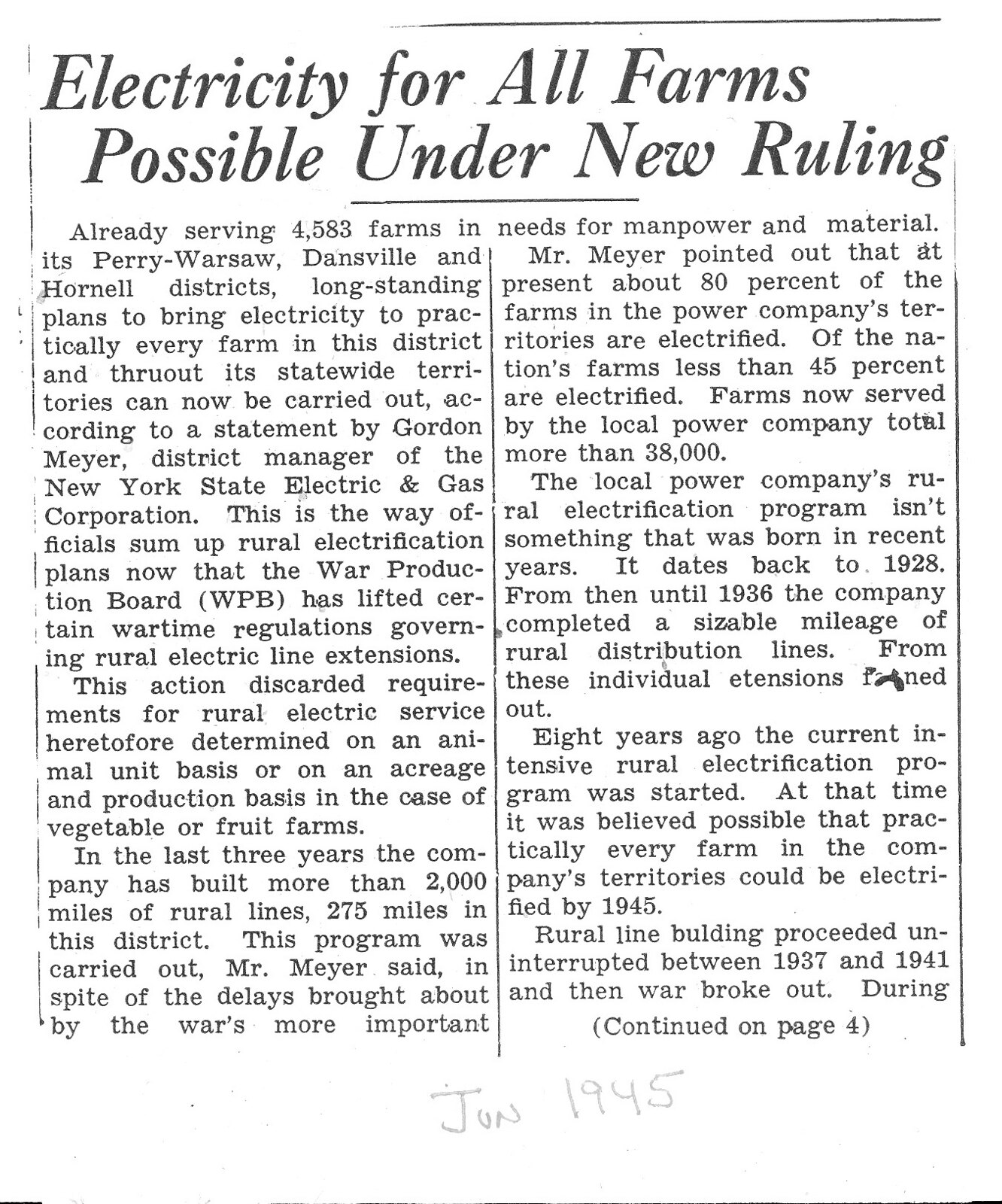This image is a scan of an old newspaper or magazine article dated June 1945, as noted in pencil at the bottom. The article is split into two columns and is titled "Electricity for All Farms Possible Under New Ruling." It states that 4,583 farms across the Perry, Warsaw, Dansville, and Hornell districts are already being served by the New York State Electric and Gas Corporation. The article elaborates on longstanding plans to extend electricity to practically every farm in the district and statewide. This expansion is now feasible due to the War Production Board lifting wartime regulations on rural electric line extensions. According to Gordon Meyer, District Manager of the corporation, the relaxed regulations will discard previous requirements for rural electric service, which were based on the number of animal units or acreage and production, particularly for vegetable or fruit farms. This period marks the transition from wartime restrictions to peacetime development priorities.